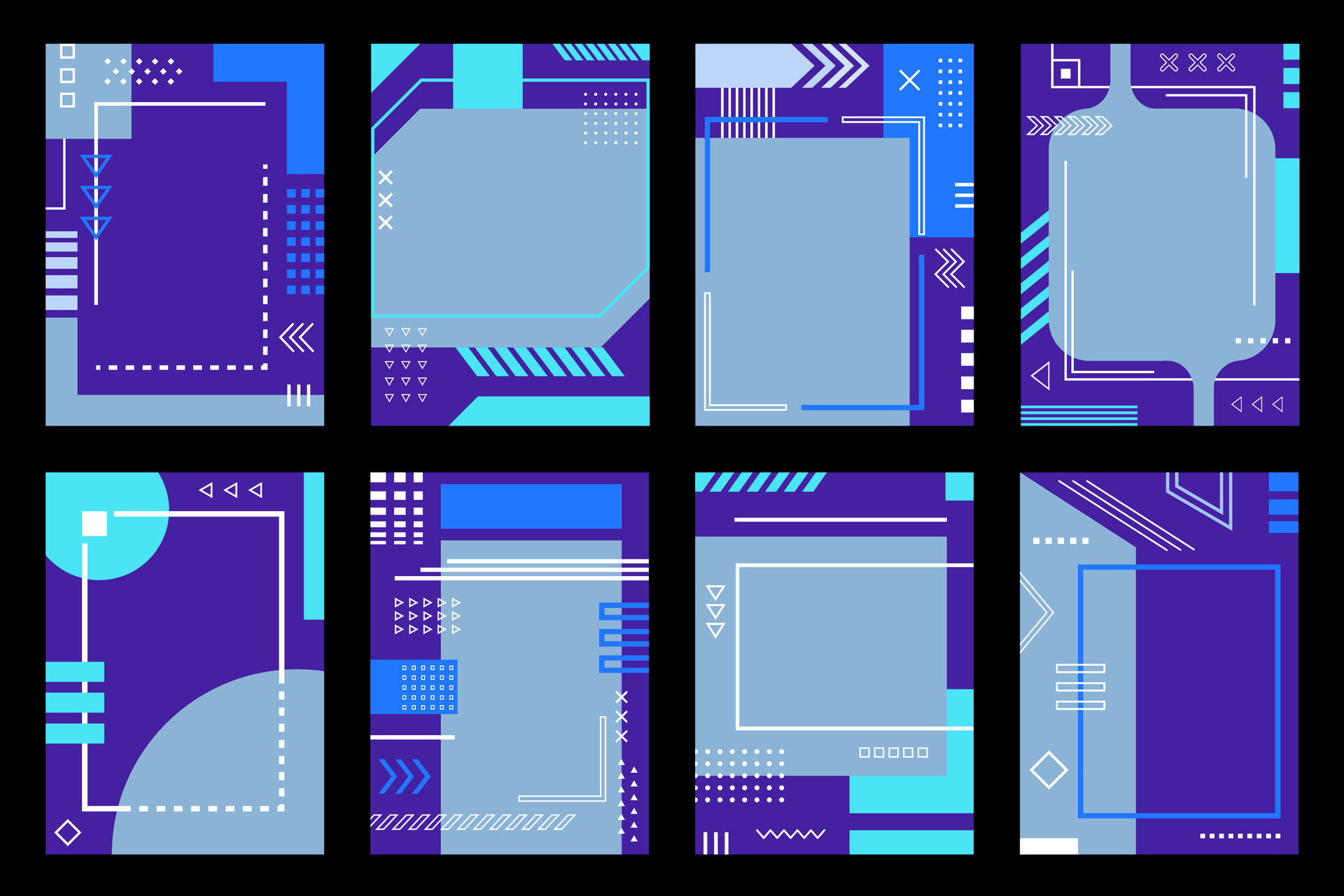The image is a poster featuring eight computer-generated designs arranged in two rows, each containing four rectangular boxes. These boxes are set against a black background and are partitioned by black lines. The designs are predominantly in dark blue, gray, and dark purples, interspersed with accents of light blue, teal, and white. Each box presents a complex geometric motif combining elements reminiscent of circuit boards and system diagrams, with intricate shapes like diamonds, crosses, triangles, and arrows. Dotted and solid lines, white arrows, and varied rectangles create a visually striking, almost technical aesthetic that evokes the feeling of a stylized computer network. Each design varies slightly, incorporating a mix of small squares, squiggly lines, and other geometric patterns, contributing to an overall impression of a high-tech schematic.